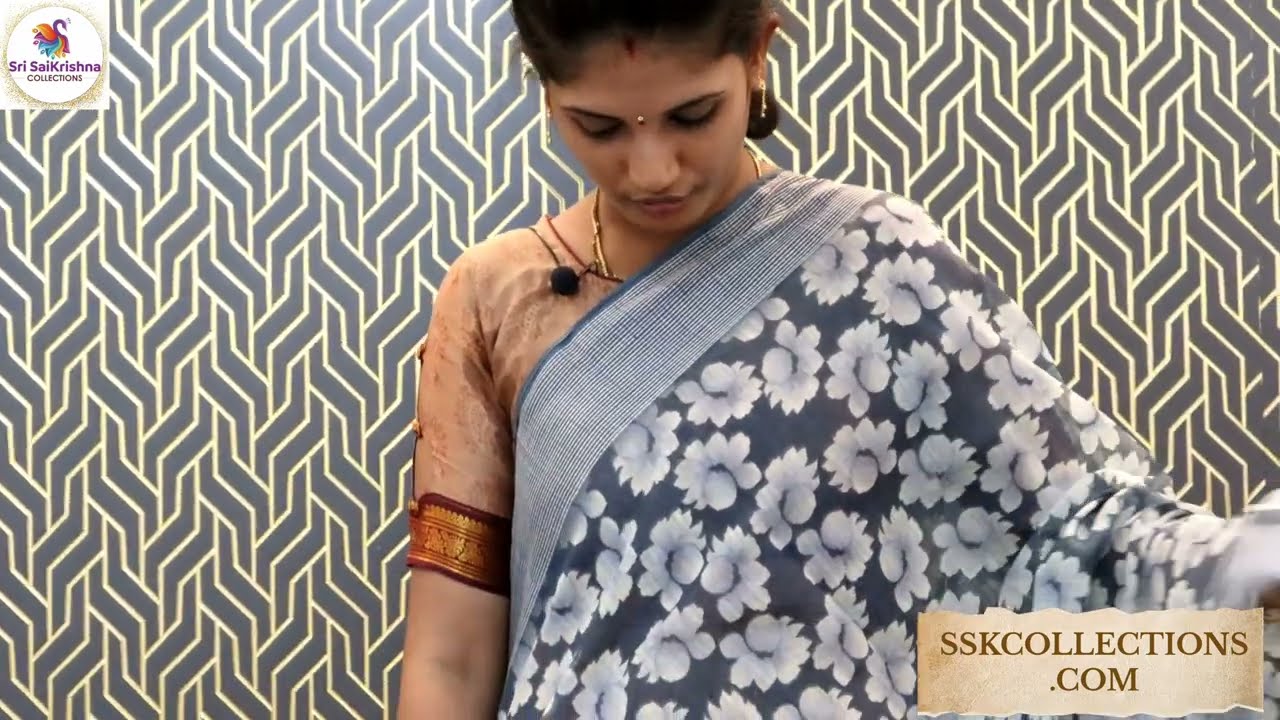A young Asian Indian woman is centered in the image, which appears to be a screenshot from a webpage. She stands against a grayish-blue abstract patterned background that has a three-dimensional stairway effect with gold borders. The woman is adorned with a decorative metal dot and a diamond-shaped medallion between her eyes. She’s dressed in a traditional Indian outfit featuring a floral-patterned sari-like cloth draped diagonally over her left shoulder and an orange t-shirt underneath. Her skin is a brown tan tone. In the bottom right corner, a rectangular text reads "sskcollections.com," while the upper left corner features a logo stating "Shree Sai Krishna Collections." The image combines muted and vibrant hues, including gray, gold, orange, red, black, and tan.